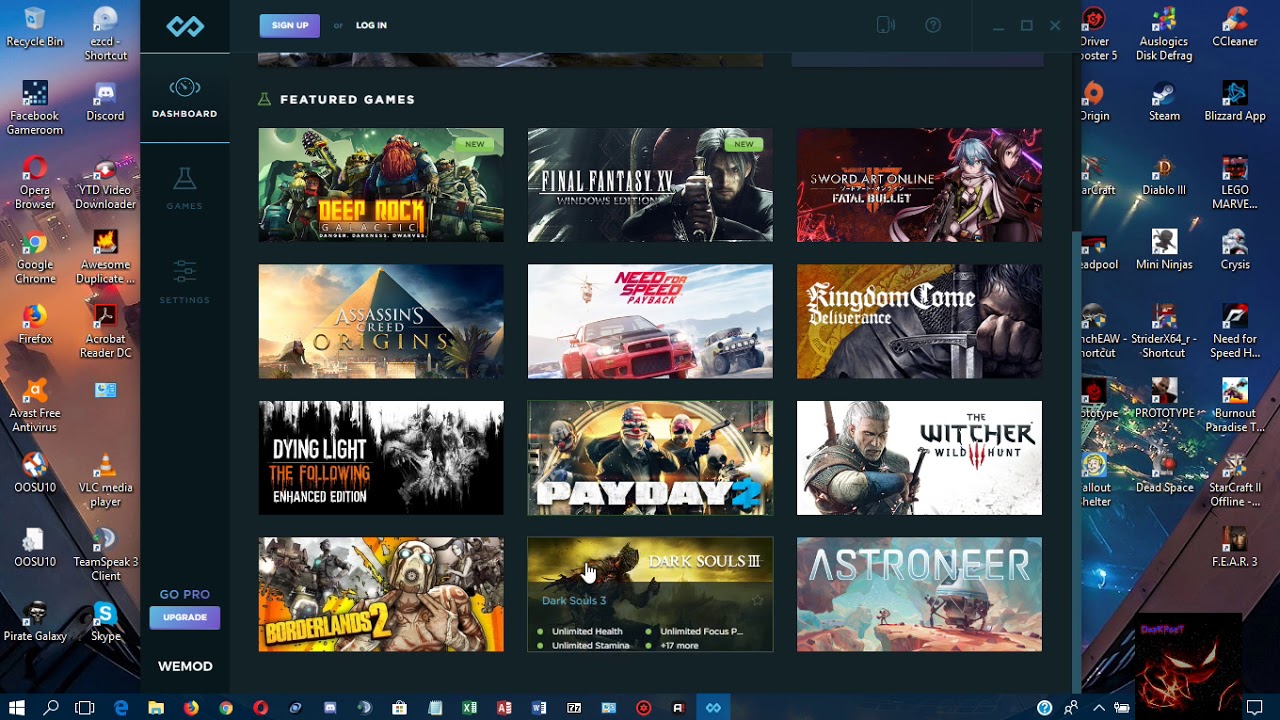This colorful horizontal screenshot captures the home screen of a desktop computer brimming with icons that engulf the entire screen. The background of the desktop features a vividly illustrated, multicolored image, adding to the visual richness.

At the bottom of the screen, the taskbar is populated with a multitude of colorful icons. Dominating the center of the screen is a gray pop-up box that resembles a gaming console interface. The top left corner of this box is marked by a blue icon mimicking an infinity symbol. Positioned next to this icon is a purple button labeled "Sign Up," and to its right, in white text, it reads "Log In."

Beneath these options, the dashboard continues downward, featuring icons labeled "Games" and "Settings." At the bottom of this section, a message reads "GoPro Upgrade" accompanied by a purple button below it. Further down, in white text, the word "WeMod" is prominently displayed.

The lower section of the pop-up box showcases a selection of 12 horizontal images, each representing different games available on this platform. Noteworthy titles among these include "Payday 2," "Astroneer," "The Witcher Wild Hunt," "Kingdom Come: Deliverance," "Dying Light: The Following Enhanced Edition," and "Borderlands 2." 

The overall scene is a vibrant and visually engaging snapshot of a dynamic and diverse gaming dashboard.